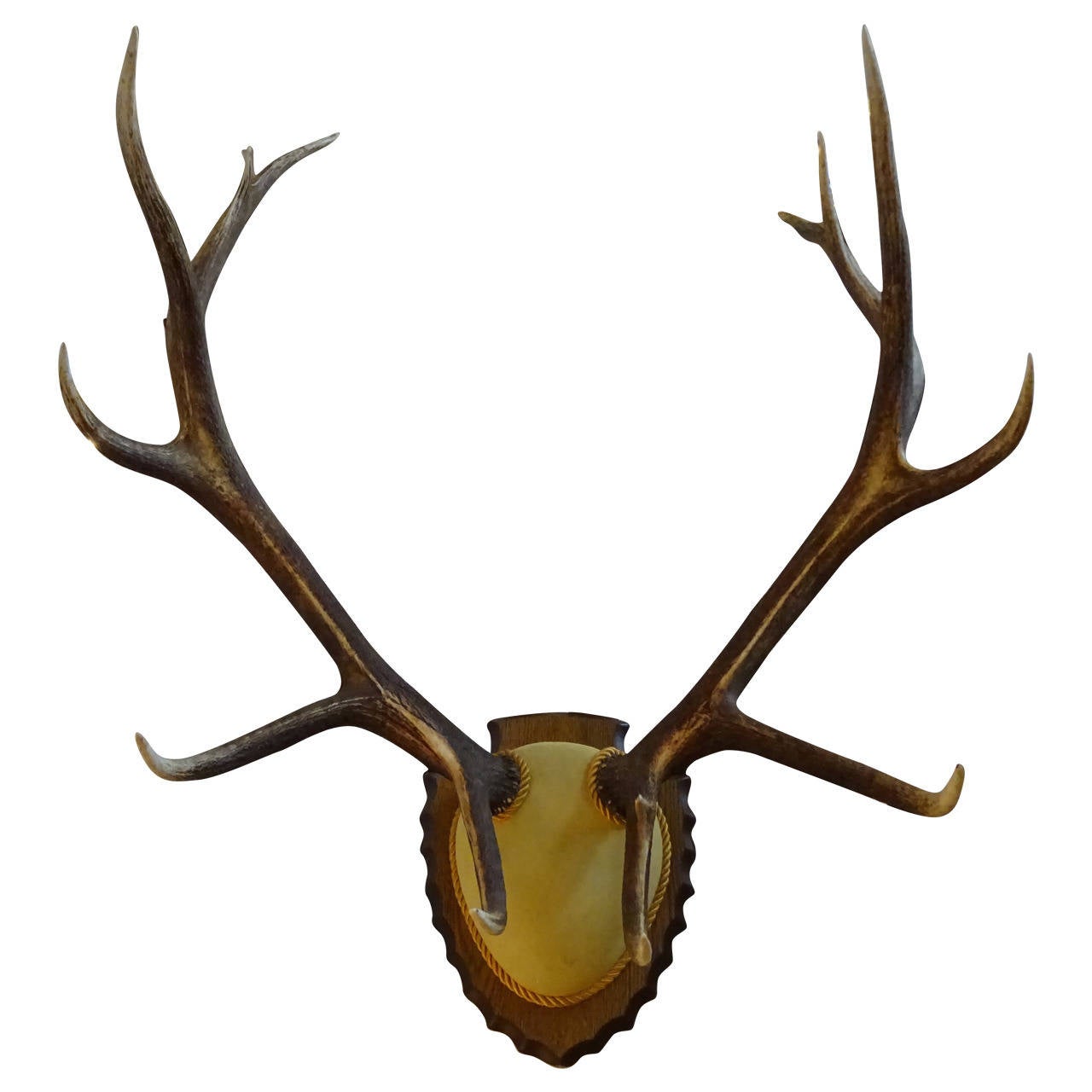The image is a staged, full-color photograph of a mounted deer trophy prominently displayed against a plain white background. The antlers, with a total of eight points, are the focal point of the image. These antlers are attached to a dark brown wooden base, intricately shaped like an upside-down stone arrow or shield, reminiscent of Native American craftsmanship. This wooden base features a secondary, golden-colored shield in the center, bordered by a rope-like design, adding a touch of elegance. The antlers themselves are long, extending upwards and outwards with branches that curve inward, varying in shades from medium to dark brown with slightly lighter tips. This striking arrangement balances both natural beauty and meticulous design.